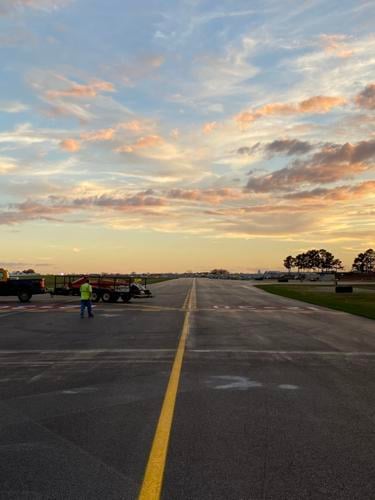This photograph captures an expansive runway or long road, distinguished by a prominent yellow line painted down its middle and additional markings throughout. The wide asphalt surface stretches far into the distance, emphasizing its considerable length and hinting more towards a runway's vast expanse than a mere street. Alongside the road, patches of grass lead to a collection of distant trees set against a sprawling sky. The sky above transitions from a clear blue at the top to shades of pink, gray, and orange closer to the horizon, suggesting the tranquil beauty of a sunset.

In the left portion of the image, a man dressed in a high-visibility neon yellow or green shirt and blue jeans is seen next to a red truck. The truck, almost out of frame, pulls a trailer carrying unidentified items, possibly red. The man appears to be walking away from the camera, further emphasizing the depth and scale of the scene. The serene yet dynamic composition highlights both the atmospheric beauty and subtle human activity in this landscape.